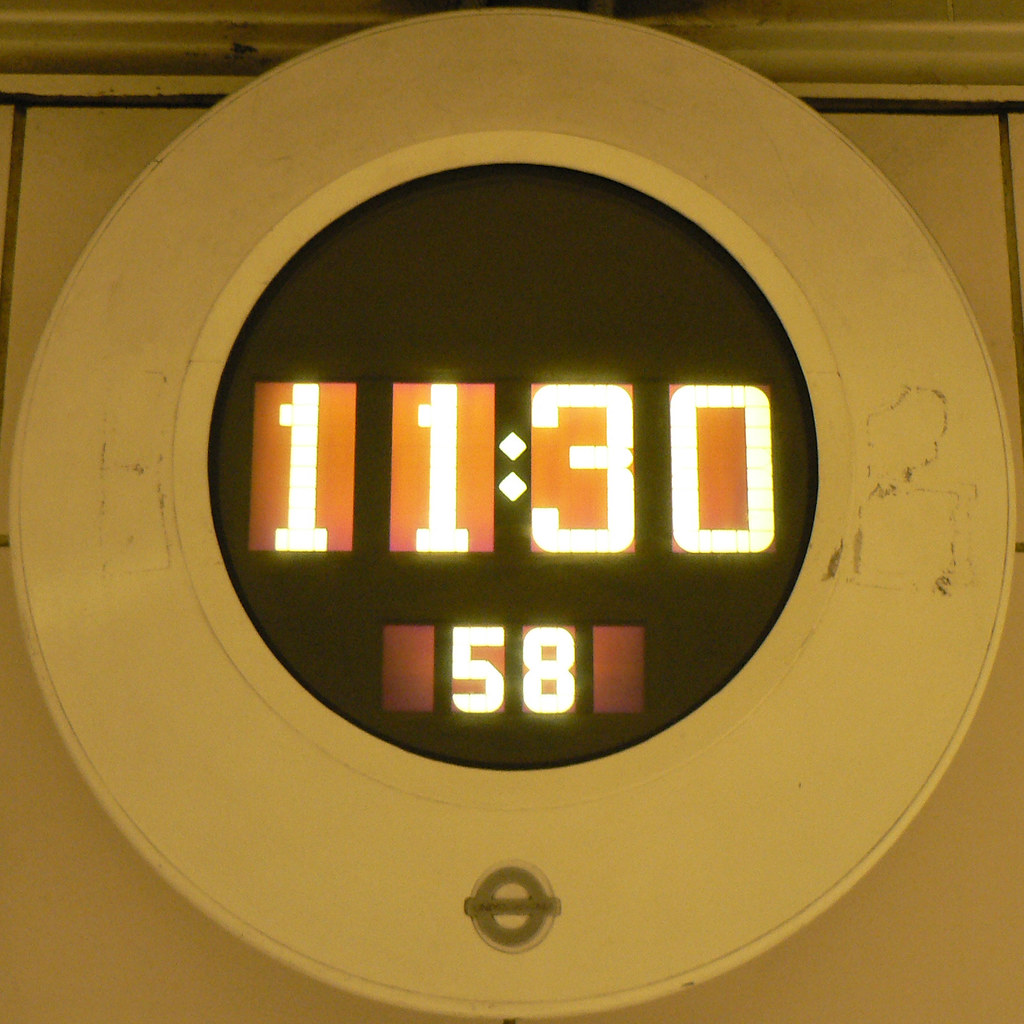This image depicts a heavily scratched gold metal wall clock with a circular design resembling a plate with the bottom cut out. The clock displays the time "11:30:58," indicating 11:30 and 58 seconds, but without specifying a.m. or p.m. The clock's face, encircled by a thick gold ring, shows a black background with bright white numbers. The intricate details include four separate rectangular segments displaying the time and additional separated segments at the bottom for the seconds. The clock is positioned centrally within the frame, filling the entire view, and is set against a similarly colored, tiled floor in light brownish or dark ecru hues. The bottom center features a distinctive circular logo with a line through it. The overall appearance is marred by considerable scratches and marks, especially on the right side, giving it a worn and dirty look.